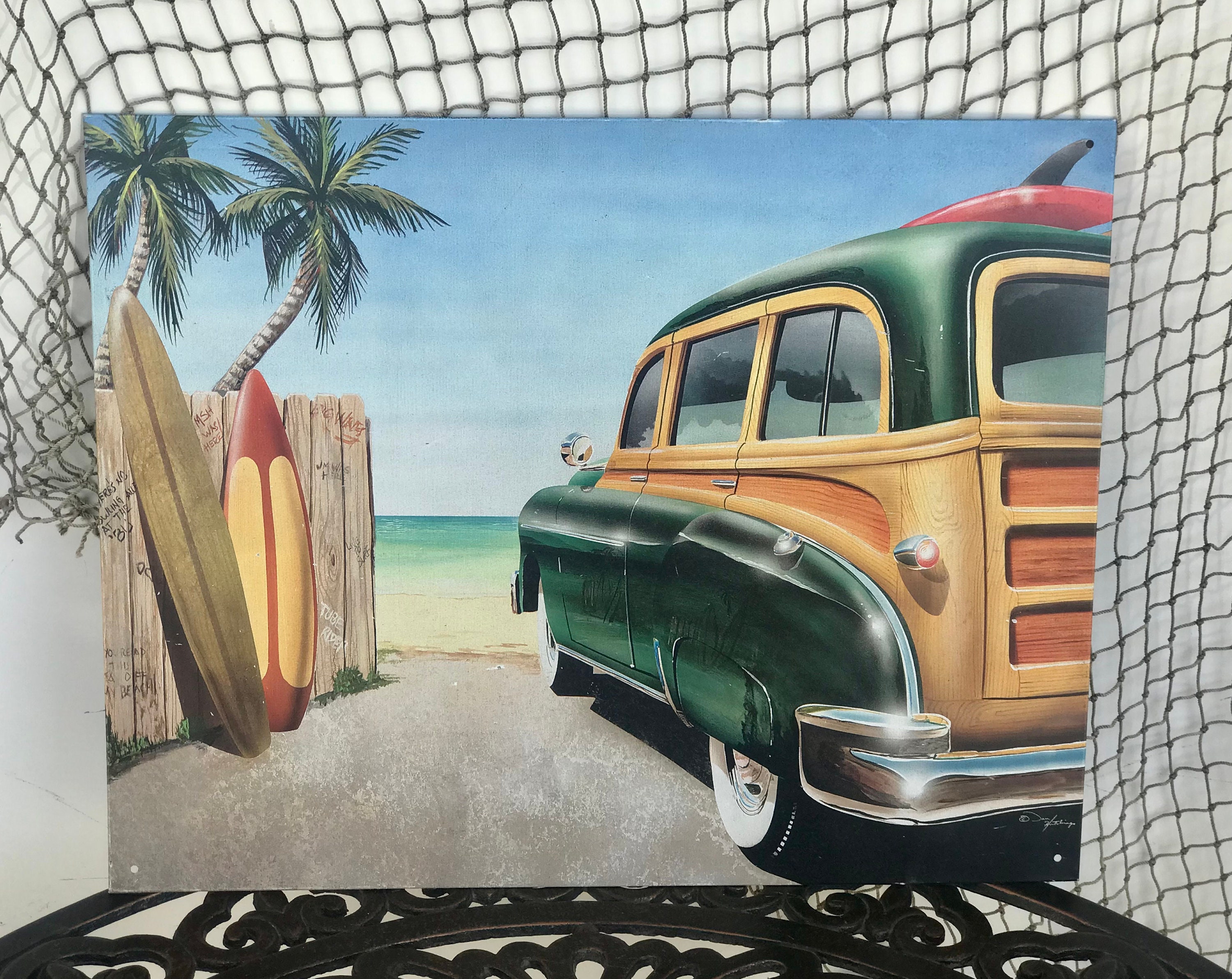The image depicts a vintage postcard pinned against a wall, with a fishing net elegantly draped behind it. The postcard features an intricate, old-fashioned 1950s-1960s station wagon. Dominantly green with wooden paneling, the car is equipped with a red surfboard, complete with a black fin, mounted on its roof. The station wagon is positioned on a beach, facing the inviting ocean waves under a clear, sunny sky. The beach scene includes two tall palm trees and a brown picket fence adorned with graffiti, situated to the right. Against the fence, two surfboards are propped up – one is long and brown, while the other is shorter with vibrant yellow and red hues. The backdrop of the entire scene is a finely patterned cast iron plate, adding a touch of vintage charm, while the surrounding environment suggests a cozy beach house setting, accentuated by the ambient shadows and sunlight.